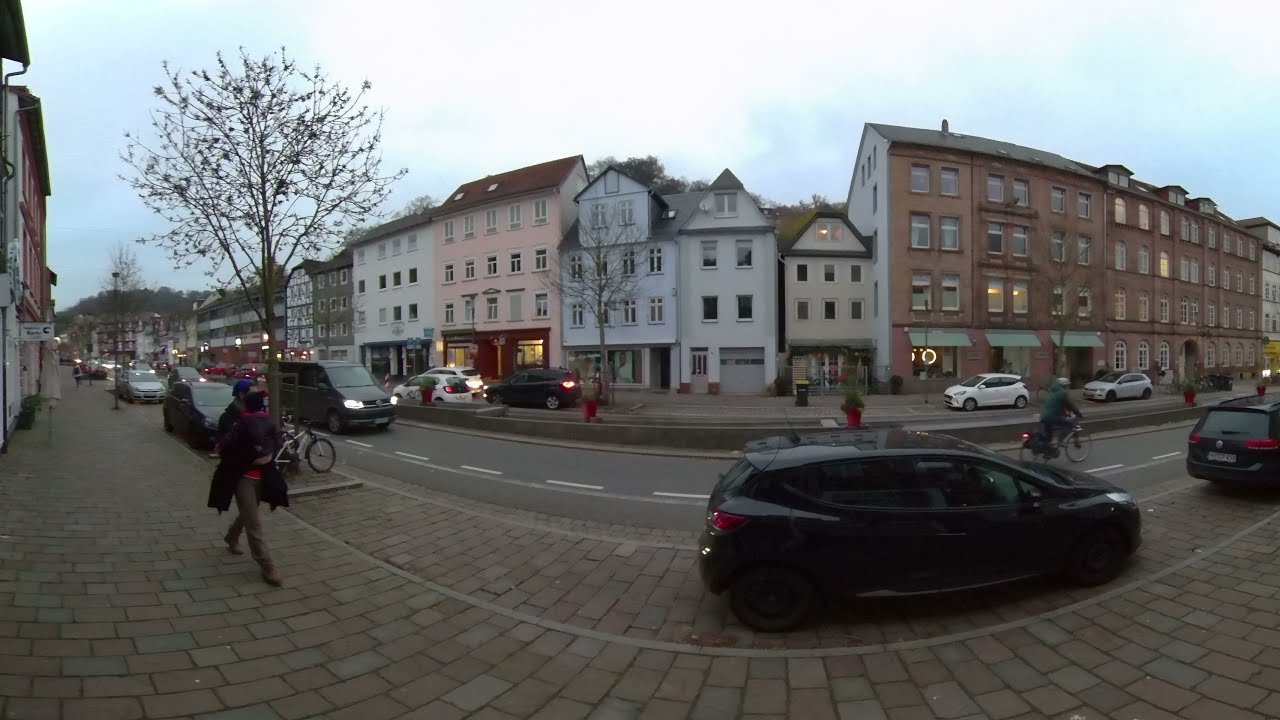The image captures a bustling European urban street scene at dusk, characterized by a cobblestone walkway and a curving row of colorful, predominantly three- to four-story row houses in shades of brown, white, pink, and tan. The street, likely four lanes wide, features a mix of parked cars and moving vehicles including vans, SUVs, and sedans. Visible on the right is a brick sidewalk with little red pots holding bushes, and in the forefront, a brick-paved parking area. Among the activity, a person rides a bike down the street, and a woman walks along the cobblestone path. The first floors of the buildings house lit-up shops, enhancing the lively atmosphere. The road itself curves elegantly, bordered by a cement center divider, emphasizing the architectural rhythm of the cityscape.